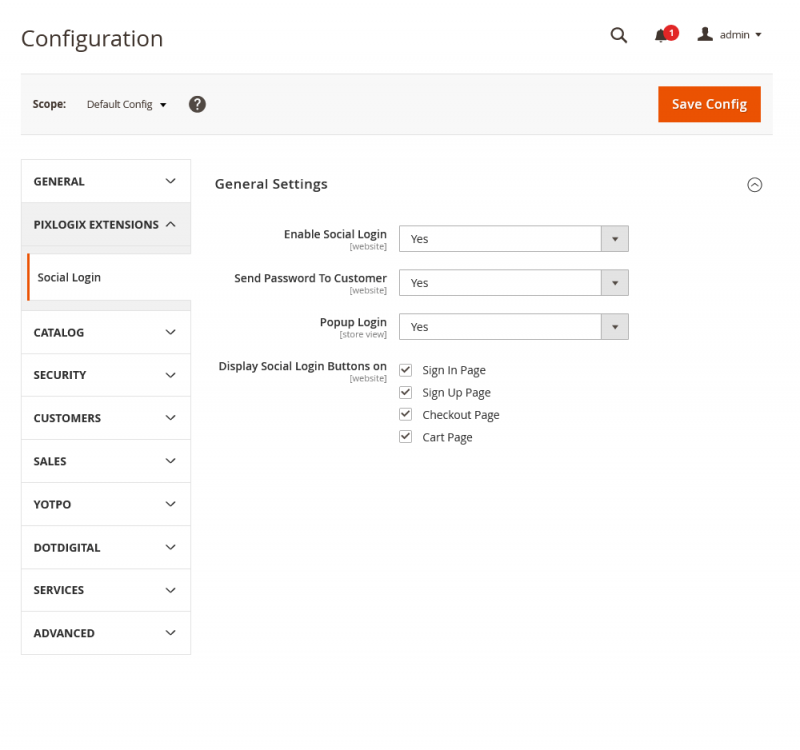**Detailed Caption:**

The image displays the configuration section of a website's administrative interface. At the top left, the header reads "Configuration," with a search magnifying glass icon, a notifications icon indicating one notification, and an admin drop-down box featuring a user icon situated to the right. Just below this header, within a light gray area, "Scope" is labeled followed by a "Default Config" option and a drop-down box, along with a help icon denoted by a question mark inside a circle. Farther to the right is a prominent orange "Save Config" button.

Below this header is a left sidebar designed for navigation. It includes a series of expandable menus: "General" with a drop-down arrow, "PIXLOGICS Extensions" with a drop-down arrow (currently expanded), and sub-sections including "Social Log-in." Continuously listed in a vertical fashion are other categories with drop-down arrows: "Catalog," "Security," "Customers," "Sales," "YOTPO," "Services," and "Advanced."

To the right of the sidebar, the page displays "General Settings." The first setting is "Enable Social Log-in" with an adjacent drop-down box set to "Yes." Following this is "Send Password to Customer" with another "Yes" drop-down box, "Pop-up Log-in" featuring the same "Yes" drop-down, and finally "Display Social Log-in Buttons On." Beneath this last option, it lists "Website" and four checked checkboxes for "Sign-in Page," "Sign-up Page," "Checkout Page," and "Cart Page."